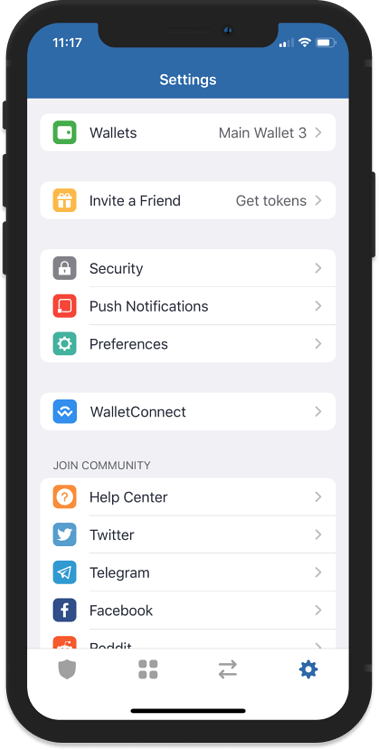The image depicts the settings screen of what appears to be a modified Android operating system, possibly unique to Samsung. The interface, diverging from traditional Android layouts, features a white background with a somewhat outdated design. Various menu options are listed, including "Settings," "Wallets," "Invite a Friend," "Security," "Push Notifications," "Preferences," "Wallet Connect," "Help Center," "Twitter," "Telegram," "Facebook," and "Reddit."

The "Wallets" section indicates "Main Wallet 3," though it's unclear whether this denotes the presence of three wallets or a previous deletion of two. Adjacent to "Invite a Friend" is a button labeled "Get Tokens," the function of which is unspecified. Towards the bottom of the screen, there are additional icons whose purposes aren't immediately clear: a shield icon, a grid icon, and one with two arrows pointing left and right.